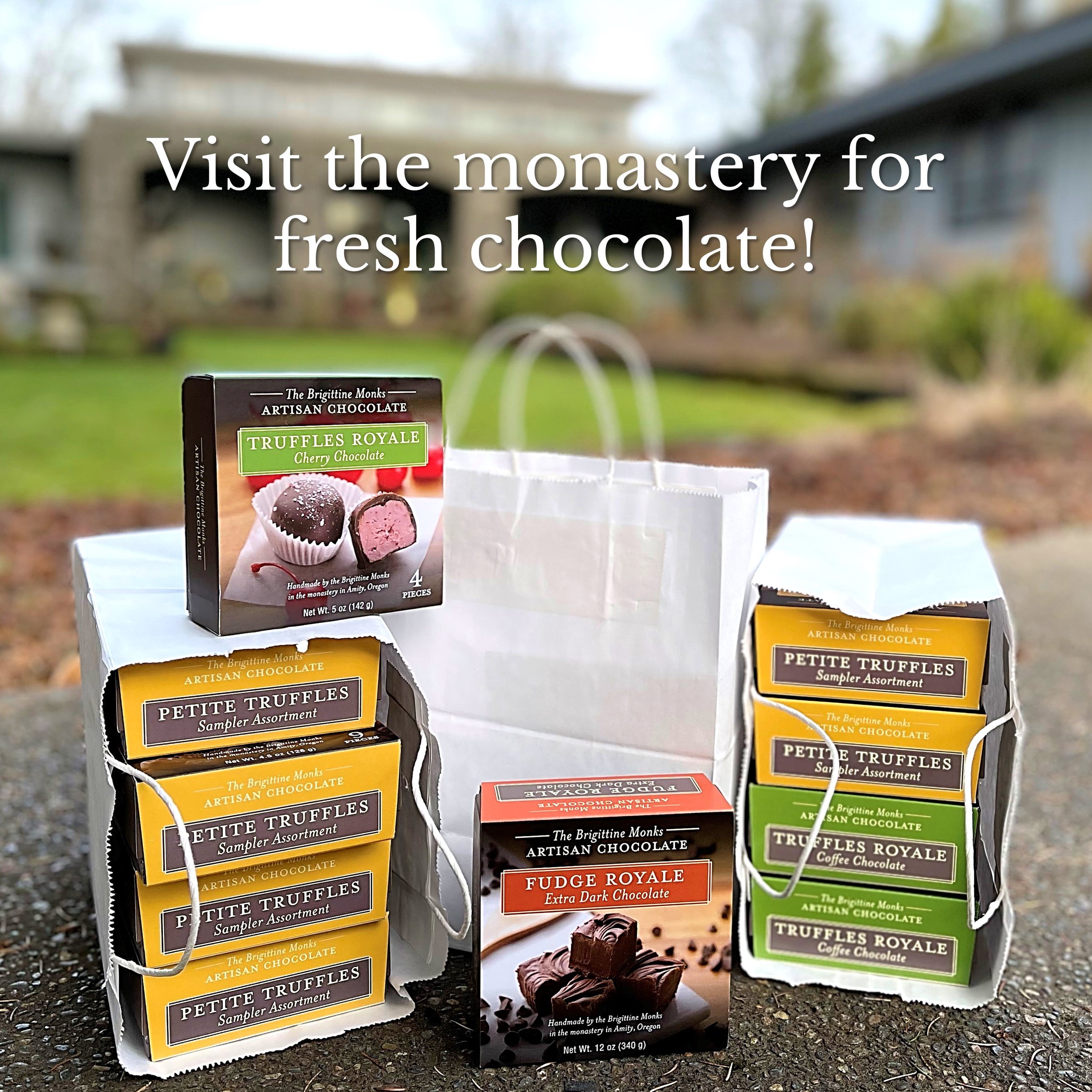This image showcases an enticing assortment of artisanal chocolates displayed on a sidewalk in front of a slightly out-of-focus building with green grass in the background. At the top of the photo, text reads, "Visit the Monastery for Fresh Chocolate," inviting viewers to explore these monastic delicacies. The chocolates, crafted by the Bridgetine Monks, are housed in a variety of colorful boxes and white paper shopping bags with handles. 

Key items include boxes labeled "The Bridgetine Monks Artisan Chocolate," with specific products like "Truffles Royale Cherry Chocolate" containing four pieces, and "Fudge Royale Extra Dark Chocolate." The assortment also features multiple "Petite Truffles Sampler Assortment" boxes, some in yellow and others in green, and "Truffles Royale Coffee Chocolate." Three white bags are present: two bags each holding four boxes of truffles side by side, with one bag’s contents obscured as it is arched upwards. The colors of the boxes range from dark orange or light red to green and yellow, creating a vibrant and mouth-watering display of monk-made chocolates.